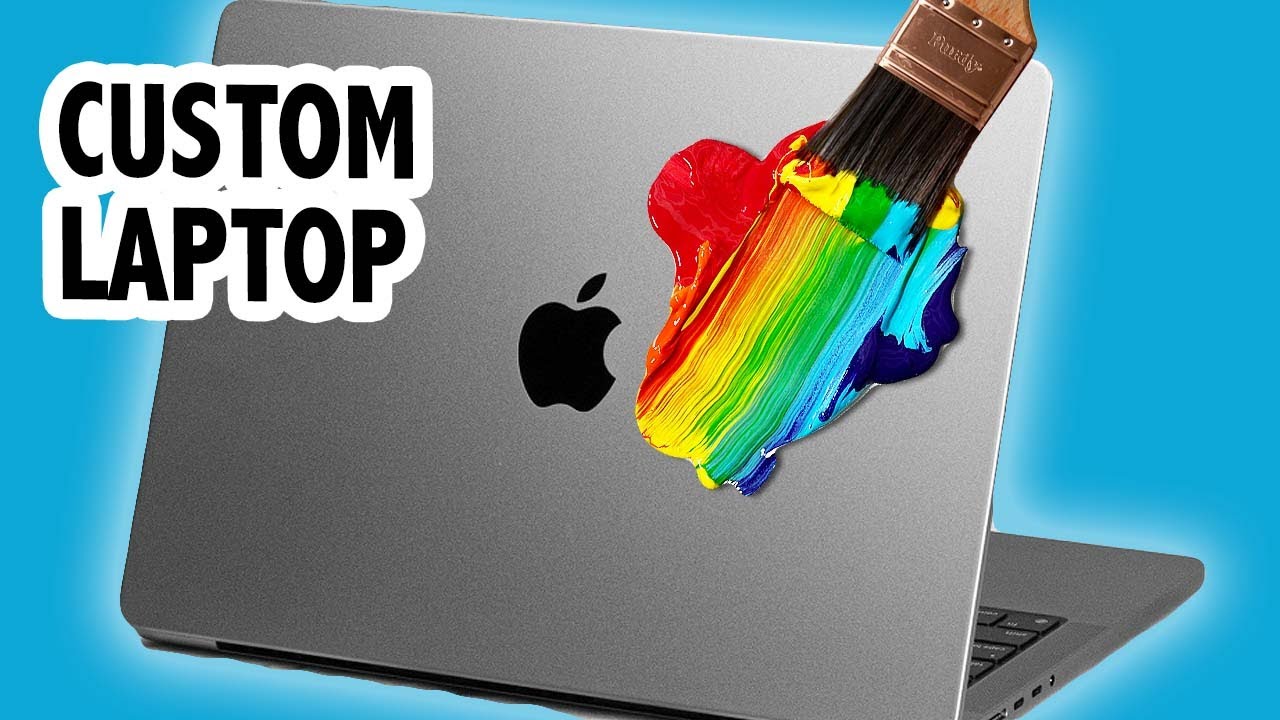The image appears to be a computer-generated advertisement possibly from YouTube, featuring a MacBook standing upright against a vivid robin's egg blue background with a highlighted glow surrounding the laptop. The silver MacBook is open, prominently displaying the black Apple logo at the center. To the top left of the laptop, bold black uppercase letters with a thick white border spell out "CUSTOM LAPTOP." On the lid of the MacBook, a bronze wooden paintbrush with rainbow paint—consisting of red, orange, yellow, green, light blue, and dark blue hues—is depicted, creating a streak of paint across the surface. The brush appears to be in motion, pushing through a large splotch of vibrant colors that extends from the top right to the left side of the laptop lid. The overall impression of the image hints at a somewhat amateur editing job, evident from the uneven edges and a slight white corner that was not fully integrated into the blue background.